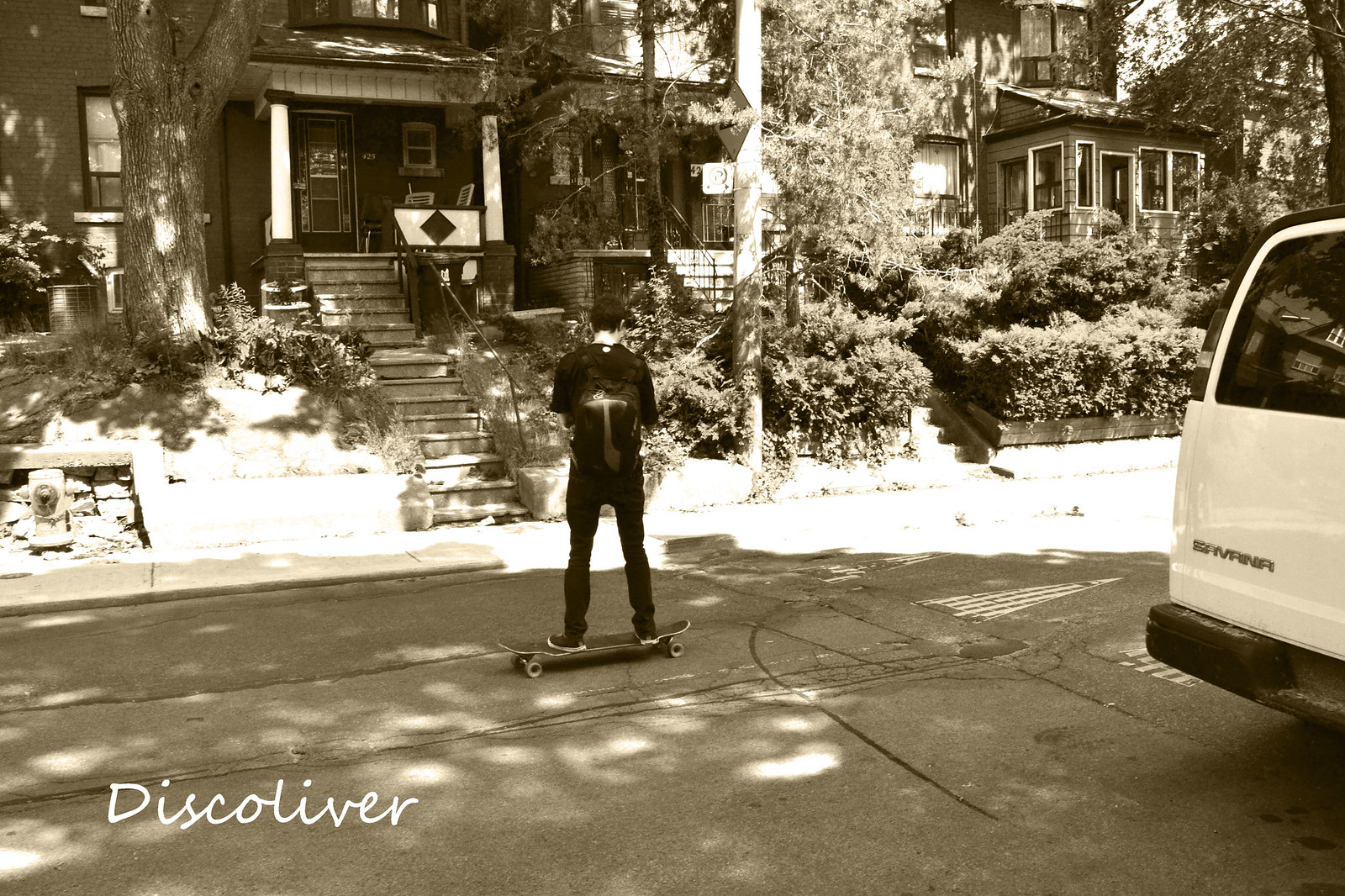In this black and white photograph by Disk Oliver, a 15-year-old boy is captured momentarily still on his skateboard. The image appears to have a sepia tone, lending it an old-fashioned, high-contrast aesthetic. The boy, seen from behind, wears a black shirt, black pants, a black backpack, and has short black hair. He stands on a cement road adorned with white drawings, in a residential area featuring mid-century style homes. A large house with an old stairwell and columns is partially visible, along with a big tree providing ample foliage. Sunlight illuminates part of the street and faintly touches the boy, who is mostly in the shadow. In the bottom left corner, the photographer's name, "Disk Oliver," is written in minimalist cursive font.